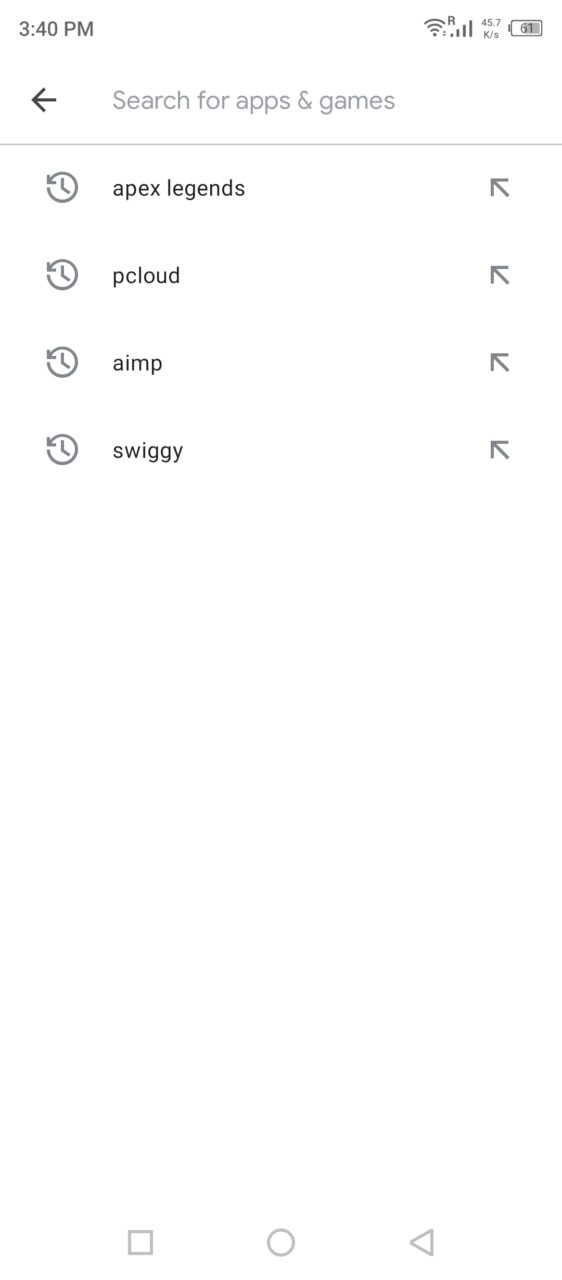This image is a screenshot of a user interface with very minimal content. At the top left, the time is displayed as 3:40 PM, alongside indicators showing a strong Wi-Fi connection with four bars and a battery level indicator. Directly below this, there is a back arrow, followed by the text "Search for apps and games" embedded within a gray search bar. The background of the entire screen is a stark, clean white, providing a very sparse look.

Beneath the search bar are four lines, each featuring a small clock icon on the left and an upward-diagonally pointing arrow icon on the right. The listed items are "Apex Legends," "PCloud," "AIMP," and "SWIGGY." The layout is symmetrical for all four items with identical icons flanking the text.

The remainder of the screen is predominantly empty, with a significant amount of white space extending to the bottom. At the very bottom of the screen, there is a row of three icons: a gray square, a gray outline of a square, a gray outline of a circle, and a gray outline of a triangle pointing to the left. These icons likely represent the standard navigation elements.

Overall, the image captures a moment in an app store or similar interface where the user may be browsing their recent or favored apps, though the screen's emptiness suggests it's either mid-setup or awaiting further user input.